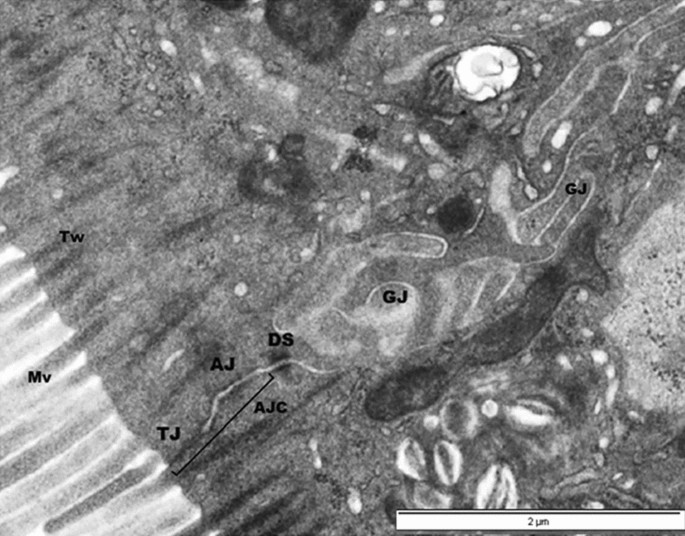The image is a detailed black-and-white microscopic photograph displaying various labeled cells within a rectangular frame, where the top and bottom sides are longer than the left and right sides. The photograph showcases a dark gray matrix speckled with smaller white dots, indicative of different cellular components. These elements are labeled with uppercase letters such as TW, MV, TJ, AJ, AJC, DS, and GJ, the latter appearing in multiple regions. In the bottom right corner, there is a white rectangle outlined in black, featuring a long black line above and centered black text that reads "2UM," serving as a scale indicator. The image's resolution is noticeably low, but the labeled sections and scale bar provide significant detail for analysis.